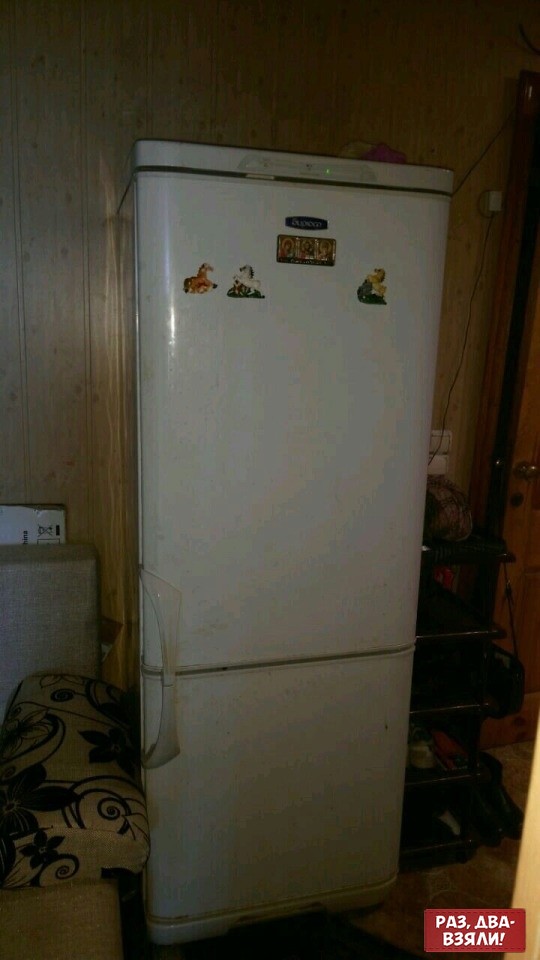This is a detailed photograph of an old-fashioned, tall white refrigerator situated in what appears to be a dimly lit kitchen or perhaps a basement room with wood-paneled walls. The fridge, showing signs of wear with slightly yellowed handles, stands prominently in the center of the image. The refrigerator has a larger top compartment and a smaller bottom freezer, both with handles on the left side. The top middle of the fridge features an unreadable logo in black with silver font. Scattered across its surface are four magnets, three depicting horses and one rectangular sticker of indeterminate detail.

To the right of the fridge, a shadowy black wire shelving unit and a door with a barely visible doorknob can be faintly made out. On the left side, an unknown white object, likely a box, rests against the wall next to a folded cardboard box and a brown cushion adorned with black floral patterns. The floor beneath the fridge shows a dark rug. This scene reflects an older, possibly rustic setting filled with miscellaneous items and a cozy, albeit slightly cluttered atmosphere.